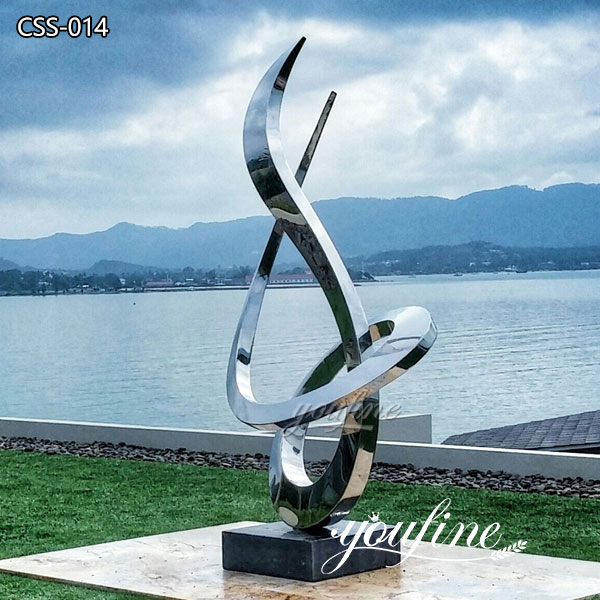This photograph captures a public artwork set beside a tranquil lake. The centerpiece is an elegant silver sculpture, approximately eight feet tall, fashioned from stainless steel and embodying a swirling, calligraphic design akin to a treble clef. The sculpture stands on a low black stone plinth amidst short green grass, with a light brown seawall delineating the waterfront. In the distance, the serene body of water stretches out, smooth and light gray, leading to a cityscape and a string of high, misty blue mountains under a cloudy sky. A few birds can be seen dotting the scene. The top left of the photograph features the text "CSS-014" outlined in black, while the bottom right corner showcases a logo reading "U-fine," where the 'U' extends into a swirl resembling a grain of wheat and the 'O' is adorned with a small crown. The entire composition is framed in shades of silver, gray, green, and a touch of light blue, creating a harmonious and reflective atmosphere.